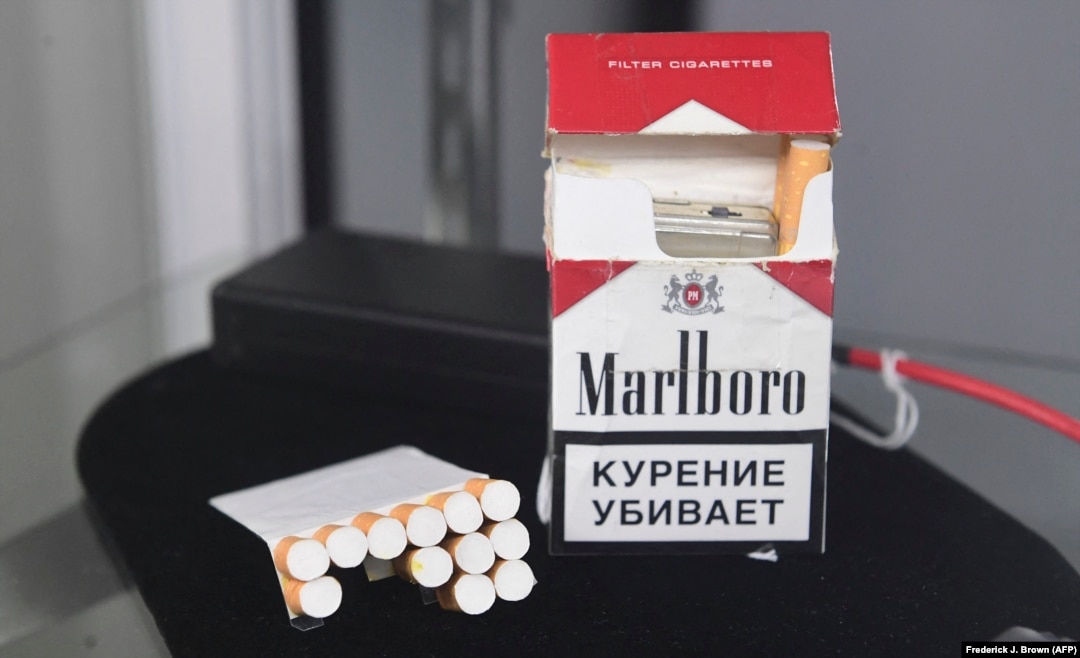This indoor photograph, rectangular in shape and approximately 6 inches wide by 3-4 inches high, prominently displays a pack of Marlboro filter cigarettes positioned on a sleek, clear glass table supported by a black column. The lower right-hand corner of the image features the credit "Frederick J. Brown (AFP)" in white text on a black background. The pack of cigarettes, with its distinctive red and white design and the text "filter cigarettes" on the lid, stands open, revealing a partial stock: two cigarettes remain alongside a silver lighter tucked inside. The bottom section of the pack displays the Marlboro branding with additional text in what appears to be Russian. To the left of the pack, the top section, removed to expose its contents, lies on the table, suggesting it has been repurposed into some sort of clandestine storage, potentially even spy gear. A cord connected to a plug is visible behind the table, hinting at a domestic or office setting.